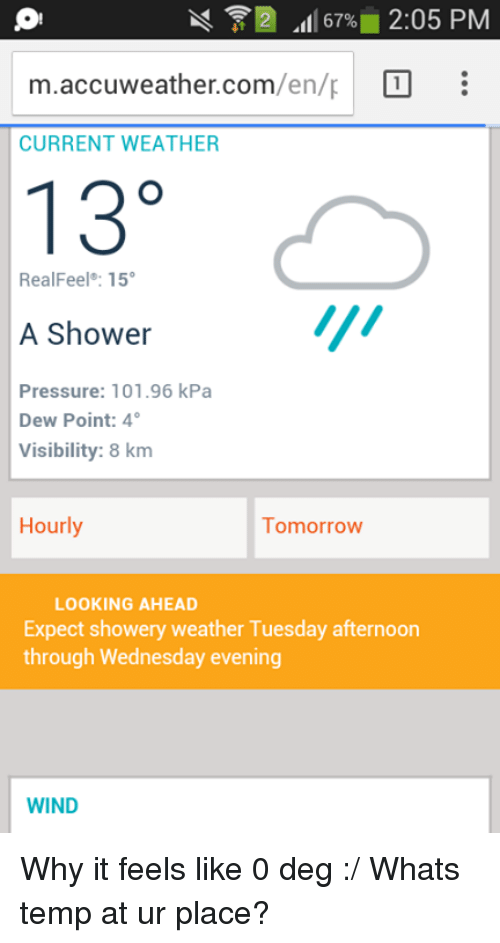On the top left corner of the black background, there is an unusual circular icon featuring an exclamation point, the purpose of which is unclear. The phone display indicates that the sound is muted, the Wi-Fi connection is strong, two web pages are open, and the battery is at 67%, highlighted in yellow. The current time, 2:05 PM, is shown in blue text.

In the browser, a white search bar with black text reads "m.accuweather.com." Only one tab is open, and three vertical dots are visible, likely for additional options. The main section of the screen is primarily white with a gray header that reads "Current Weather."

Below this, in bold black text, the temperature is listed as 13°C with a "RealFeel" of 15°C. To the right, a gray cloud icon with three blue lines indicates rain. Beneath this, in black text, the condition is described as "A shower." Additional weather details in gray text include "Pressure: 101.96 kph," "Dew Point: 4°C," and "Visibility: 8 kilometers."

Further down, two white buttons labeled "Hourly" and "Tomorrow" in greenish-orange text appear. A section with the same greenish-orange text explains, "Looking ahead, expect showery weather Tuesday afternoon through Wednesday evening." A gray bar follows, then a white bar with the word "Wind" in blue text and a black annotation saying, "Why it feels like zero degree," accompanied by a peculiar smiley face.

The message "What's temp at your place?" appears, querying someone else, noted that it is not zero degrees but actually 13°C, feeling like 15°C. Given the use of Celsius and kilometers, it is inferred that the location is using the metric system.